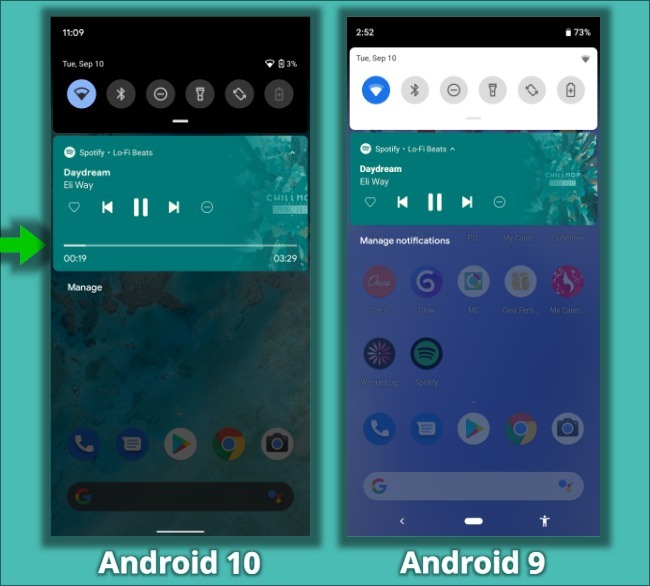The image features a serene turquoise-colored background with two cell phones placed on it. The cell phone on the left has a dark screen background displaying the time "11:09" on Tuesday, September 10th. This phone's screen is populated by numerous icons and shows a Spotify widget playing "Daydream" by Eli Way, with a progress bar indicating that 19 seconds out of the 3 minutes and 29 seconds of the song has been played. Below the widget, the word "Manage" is displayed. Along the turquoise border beneath this phone, white lettering reads "Android 10." 

An illustrative green arrow on the left edge of the image points towards this first phone, drawing attention to its details.

The second cell phone, positioned on the right, shows the time "2:52" and a battery level of 73%. Similar to the first phone, its screen also displays a Spotify widget playing "Daydream" by Eli Way, but without a visible progress bar. The word "Manage" appears under the widget, followed by "Notifications." Below this phone, white lettering on the turquoise border indicates "Android 9."

The image is devoid of people, animals, plants, flowers, or trees, focusing solely on the devices against the minimalist background.